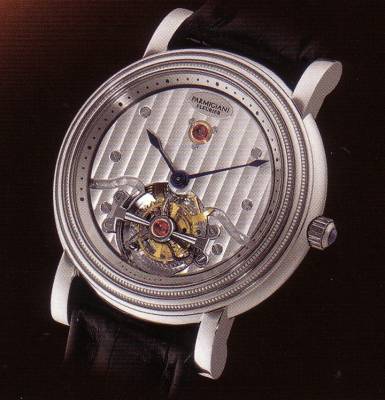In the image, we see a stunning, luxurious Parmigiani Fleurier watch against a black background. The exotic timepiece features a polished silver housing and a sleek, black strap that subtly disappears into the backdrop. The watch's intricate internal mechanisms are partially visible through a round aperture on the bottom half of the face, showcasing a sophisticated spring and gear system. The timepiece is oriented diagonally, facing towards the left. It is adorned with elegant dark blue hour and minute hands, while lacking a second hand. At the top of the watch, a small red jewel adds a touch of opulence, accompanied by a nameplate bearing the Parmigiani Fleurier inscription. The wind-up mechanism is located to the right of the watch. The luxurious design and detailed craftsmanship highlight its exotic and expensive nature, presented beautifully against the black background.